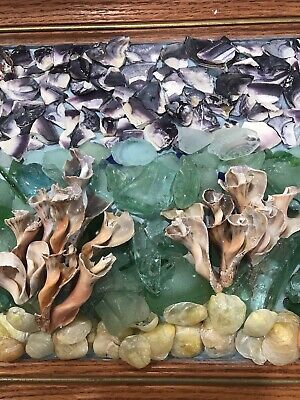This detailed 3D artwork presents an abstract yet captivating underwater scene. Enclosed within a dark wooden frame with subtle engraved stripes, the composition skillfully mimics the vibrant depths of the ocean. The bottom part of the artwork features a bed of beige, tan, and white rocks meticulously positioned to reflect the seabed. Above this, diverse green and teal elements, with hues that shimmer like glass, evoke the fluid essence of water. Twisty cylindrical formations resembling coral trees rise gracefully, presenting a burst of textures and colors, from light to medium greens. The top section of the artwork transitions into a grayscale depiction of churning bubbles and waves, suggesting the dynamic surface of the ocean. Interspersed throughout are shells and crystal-like blue elements, enriching the scene with additional depth and realism. The entire piece, anchored by its dark cherry wood frame, offers a beautifully layered and textured visual experience, masterfully blending elements to create a dynamic underwater tableau.